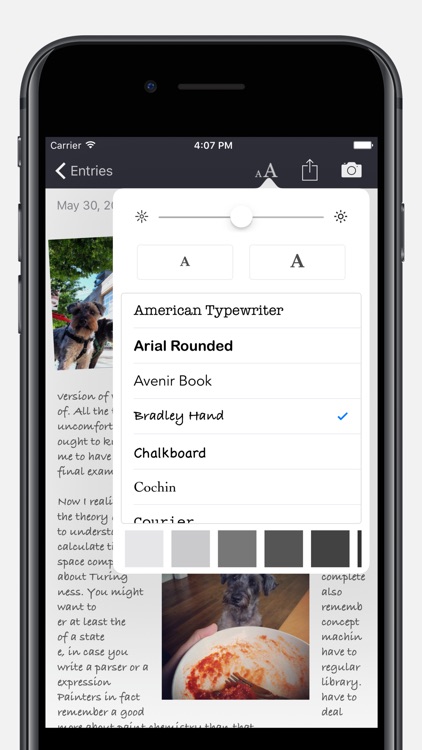The image features an iPhone with its screen on, displaying a reading app that has an open book or magazine. The view is mostly obscured by font settings, where options such as font size, type, and brightness adjustments are available. The font is set to "Bradley Hand," a lighthearted cursive style, which is evident in the partially visible text. The obstructed text hints at content related to painting, though it’s mostly unreadable and could potentially be placeholder text for app development. Additionally, the screen displays a picture of a dirty plate with spaghetti sauce and a dog.